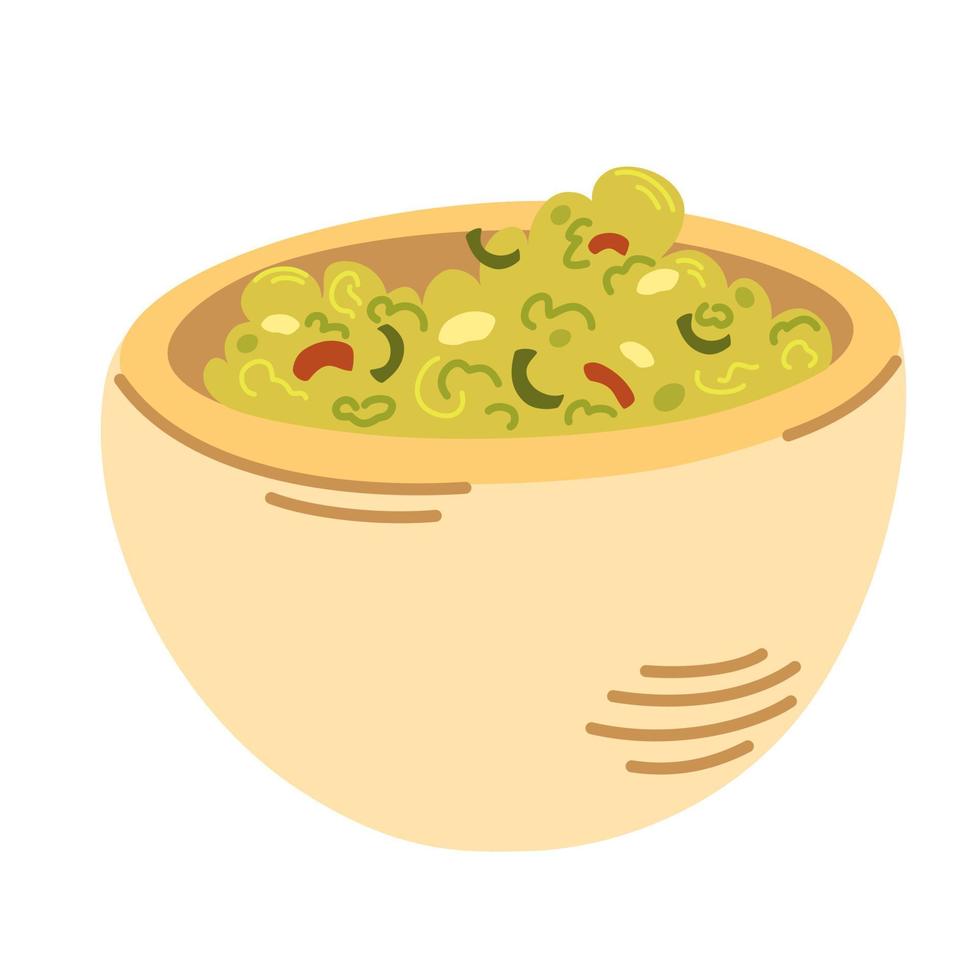This image is a color illustration with a simplistic, cartoony feel, similar to what you'd see in a children's book. It features a beige bowl set against a white background. The bowl, depicted with a tapered shape that is wider at the top and narrows toward the bottom, has medium brown lines accentuating its circular form. The top rim is colored in a peach or light golden brown shade. Inside, the bowl has a brown hue and contains a piled-up, light green substance resembling guacamole or a similar dip, curvy and not flat, with small bubbles. Scattered throughout the green mixture are bits of vegetables in red, green, white, and yellow hues, including darker green squiggly and curved lines, reminiscent of different ingredients. The overall style presents a whimsical, illustrated look where the subject appears to be floating on a white background.